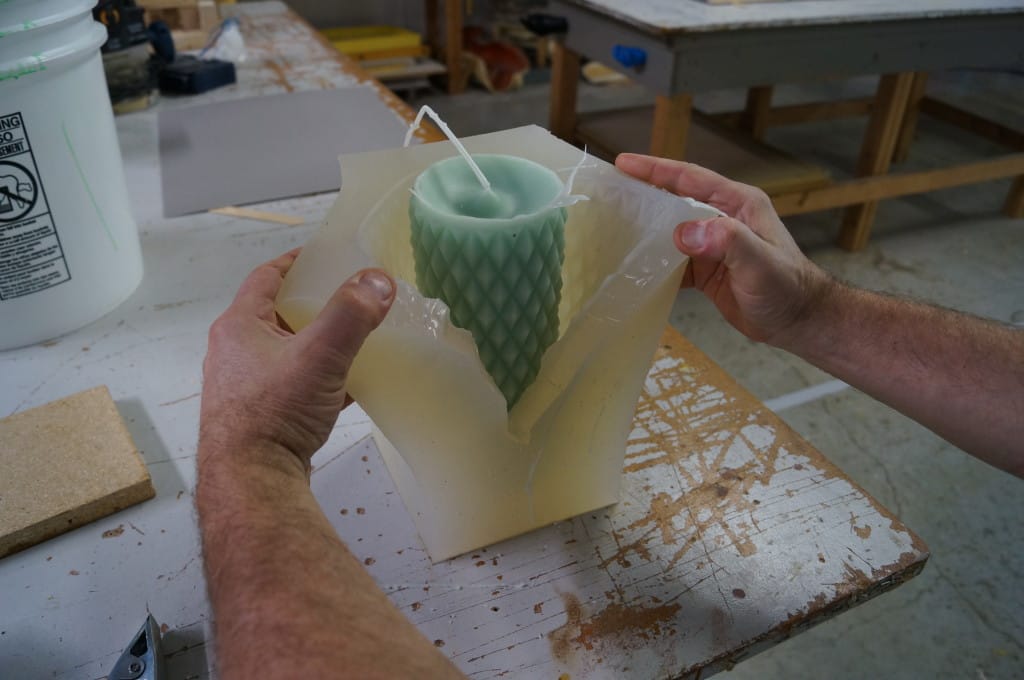In a rustic workshop setting, a man is meticulously dismantling a wax mold to reveal a beautifully crafted green candle. The cylindrical candle, adorned with a pattern of interlinked diamonds, sits prominently on a well-worn white work table, indicative of extensive use. The original mold, a waxy off-white enclosure, is being pried apart by the man's strong, hairy arms, his fingers displaying palpable effort. The candle features a long white wick, emerging from its top. Surrounding this scene are various tools and materials, including a prominent bucket to the left, seeping green goo, likely used in the candle-making process, hinting at the creation’s origin. In the background, a secondary work table adds depth to the workspace ambiance.